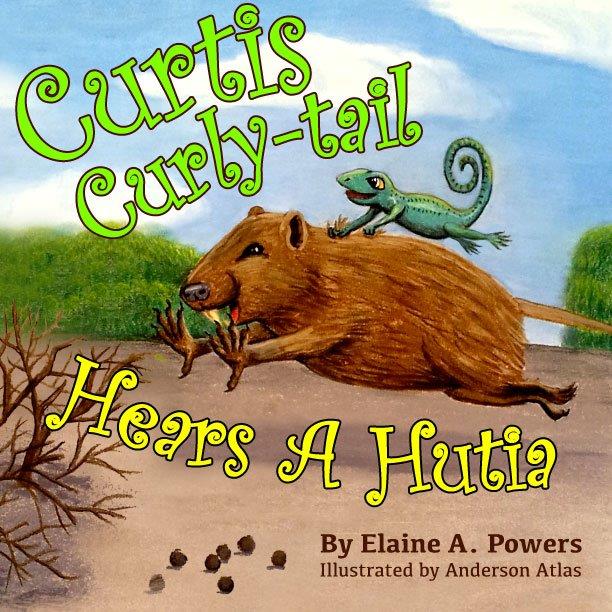The cover of this colorful children's book features a playful and lively scene. The title "Curtis Curly Tail" is written in green cursive writing, and directly below it in yellow cursive, it reads "Here's a Hootia." At the bottom, in plain text, it states, "By Elaine A. Powers, illustrated by Anderson Atlas." Dominating the center of the cover is a joyful brown rodent, energetically running across a patch of brown ground. Clinging to its back is a green lizard, identifiable by its green color with black specks in a pattern and a notably curly tail. Both animals appear happy, with open mouths that look like they are smiling. Surrounding them, the background shows green vegetation and a vibrant blue sky scattered with clouds, adding to the whimsical and humorous atmosphere of the illustration. The scene also includes some brown round objects and a dead wooden bush, enhancing the playful and not strictly realistic depiction.